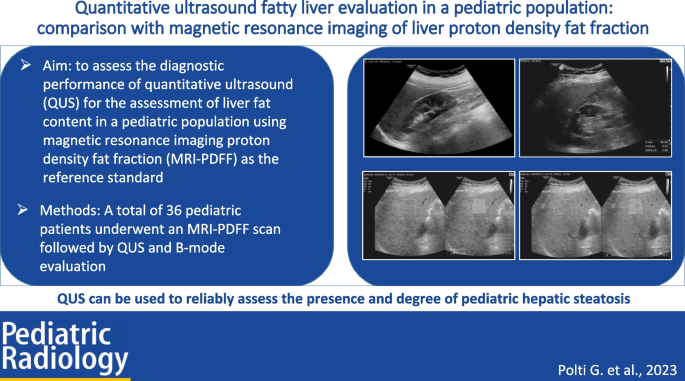This detailed image, likely extracted from a scientific study, appears instructional and suited for educational resources like textbooks or academic websites. At the top, the image is titled "Quantitative Ultrasound Fatty Liver Evaluation in a Pediatric Population: Comparison with Magnetic Resonance Imaging of Liver Proton Density Fat Fraction." Directly below this title, on the left, there is a rounded blue square detailing the aim to "Assess the Diagnostic Performance of Quantitative Ultrasound for the Assessment of Liver Fat Content in a Pediatric Population using Magnetic Resonance Imaging Proton Density Fat Fraction (MRI-PDFF) as the reference standard." To the right of this description are four small black and white ultrasound images, likely depicting varying degrees of liver fat content. The bottom of the image features a blue banner where "Pediatric Radiology" is displayed on the left, and the citation "Pulte G. et al. 2023" is listed on the right, suggesting the journal and authors of the study.